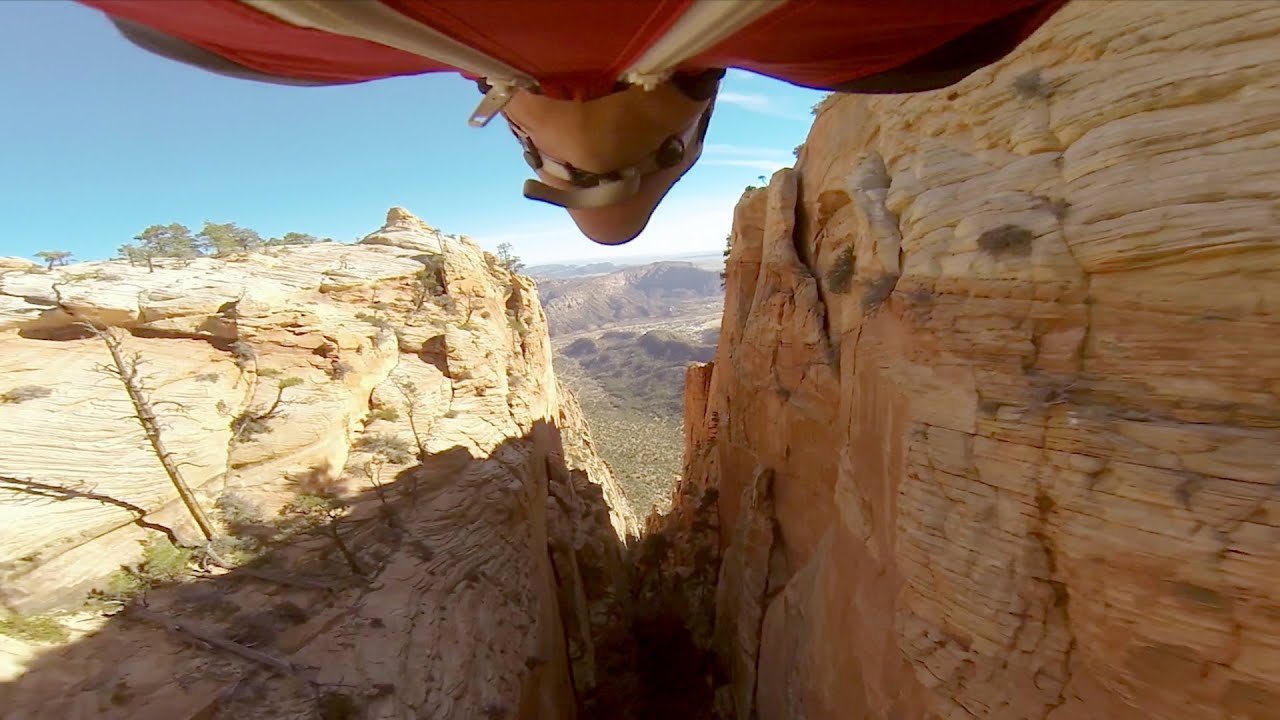In this captivating horizontal photograph, a person is captured gliding through a dramatic mountain pass or canyon, navigating an opening flanked by two imposing cliff faces. The landscape below reveals a rugged, desert-like terrain dotted with scattered green shrubs. The individual is wearing a distinctive orange wingsuit adorned with two prominent white zippers that extend up to their collar, which is secured with a white chin strap. Positioned from a GoPro attached to their body, the image offers a unique vantage point: we see the person's chest and bottom half of their head, leaving their face obscured. The canyon walls on either side are rugged and textured, primarily brown with variations of light brown hues. The far end of the canyon opens up to reveal distant mountains beneath a bright blue sky. Small clusters of trees are visible along the rocky terrain and in the far background, enhancing the striking contrast between the earthy cliffs and the vibrant sky. The overall scene is a thrilling and dramatic glimpse into the adventure of wingsuit gliding.